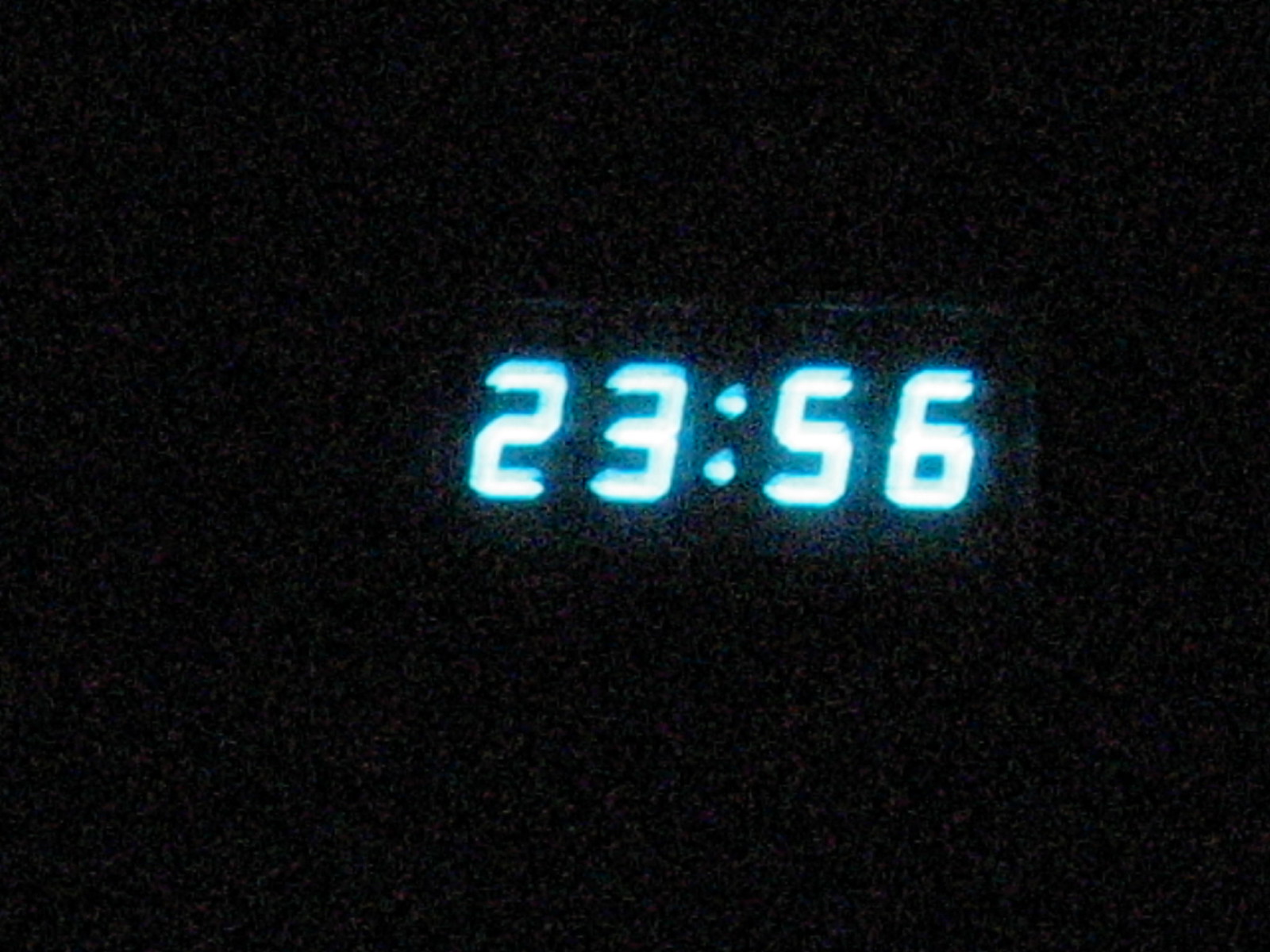This color photograph, taken at night without any auxiliary lighting, showcases a predominantly black page, save for a small section in the middle. At the center, there is a digital readout displaying the time "23:56." The digits have a striking neon effect, predominantly white with vivid medium blue edges, creating a glowing aura around each number. The image quality is compromised, appearing spotty with numerous white dots scattered throughout, indicative of inadequate lighting and the absence of proper photographic filters. The overall effect gives the impression of an image taken in suboptimal conditions, capturing a moment in the dark but with vibrant time display.